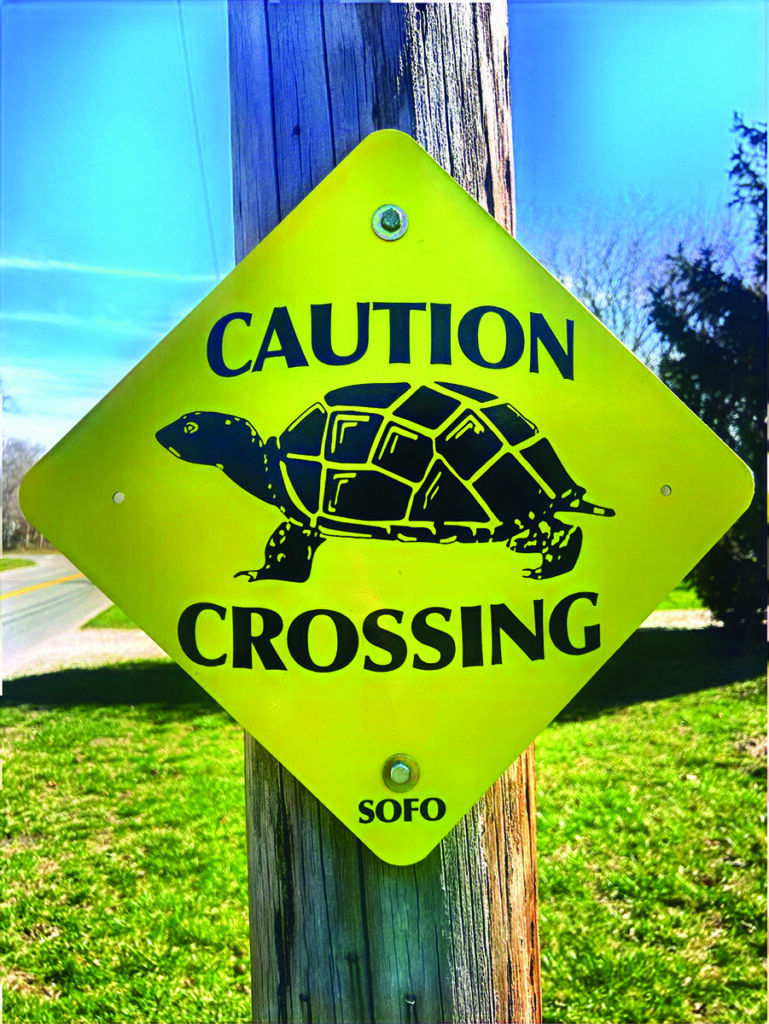The photograph captures a vividly detailed outdoor scene dominated by a thick, round wooden pole that supports a yellow, diamond-shaped street sign prominently displaying the words "CAUTION TURTLE CROSSING" in black lettering. The sign is affixed to the pole with bolts at both the top and bottom, and beneath the crossing notice is the acronym "S-O-F-O" in all capital letters. Surrounding the pole, lush, green grass stretches below while a pine tree partially enters the frame from the right side. The blue sky above is adorned with streaks of white clouds, providing a tranquil background. Additionally, the left side of the image hints at an asphalt road adorned with orange lines, enhancing the vividness of this serene yet informative setting.